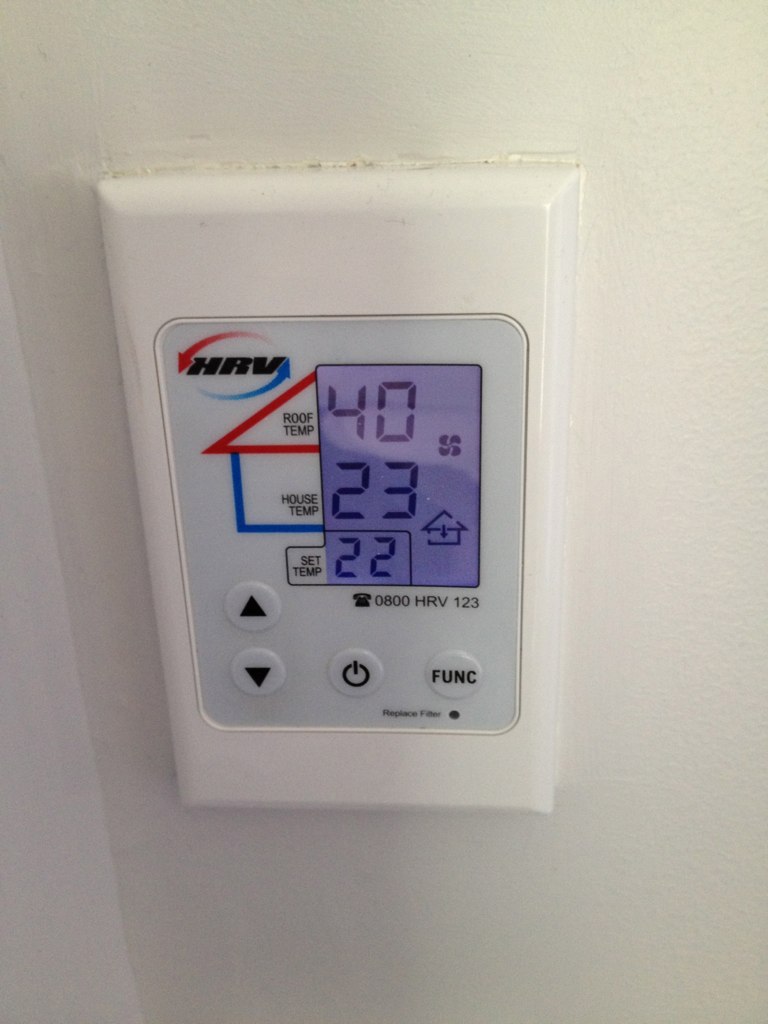This image displays a modern thermostat with an unfamiliar design, likely used in Europe as indicated by the temperature readings in Celsius. The thermostat's interface showcases three distinct temperature readings: the roof temperature, the house temperature, and the set temperature. It features two arrow buttons on the left side for adjusting the set temperature, a central button to turn the unit off, and a function button on the right side. The thermostat's casing and interface are blue, with the LED screen illuminating in a light blue hue, displaying black numbers and lettering for readability. Overall, the device appears to be a straightforward thermostat for an HVAC system.